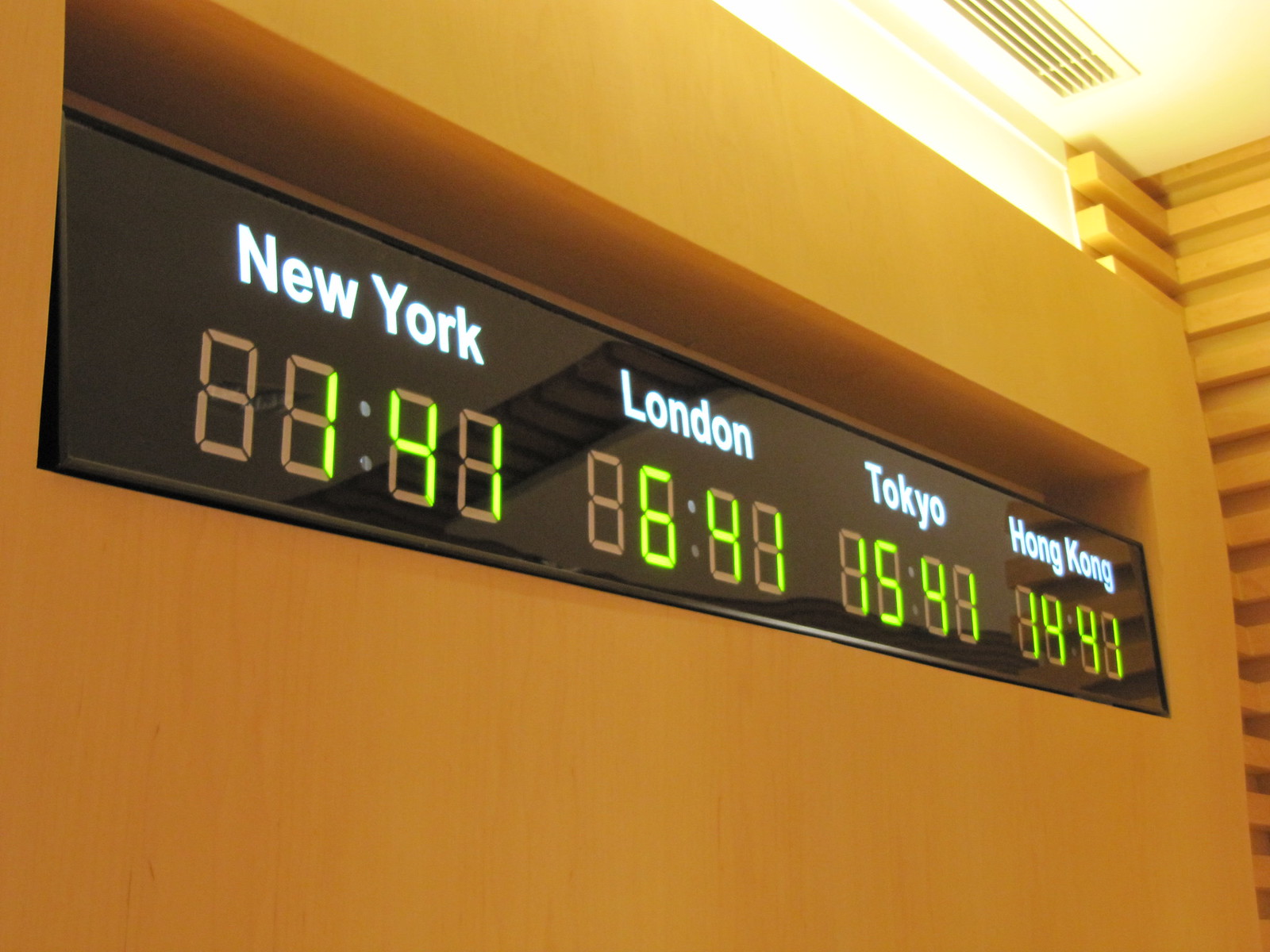This color photograph appears to have been taken at an airport and focuses on a black digital ticker embedded in a recessed beige-yellow wall. The ticker prominently displays the names of major cities—New York, London, Tokyo, and Hong Kong—with corresponding times in yellow text: 1:41 for New York, 6:41 for London, 15:41 for Tokyo, and 14:41 for Hong Kong, indicating it operates on a 24-hour clock. Above the ticker is a small window that allows natural sunlight to flood into the space, casting a warm glow on the scene. The wall also features an air duct vent on the ceiling, which is white. To the right, there's another section of the orange wall adding to the overall warm color palette. The detailed setup and background elements suggest a structured, well-lit public space, likely a part of an airport's interior architecture.